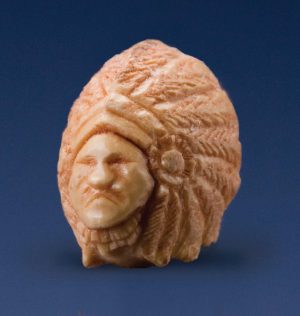The image is a square with a navy blue background, prominently featuring a carved face at its center. The carving, which occupies most of the image, gives the impression of being made out of soap, displaying a smooth, almost silky texture. The face is a brownie-tan color, evocative of a native man adorned with a large, intricate headdress that extends outward and backward, enveloping the head in a grand, flowing form. The man's facial features include a pronounced nose, a mustache, a frowning mouth, small eyes, and subtle eyebrows. Additional detail includes a floral-like element on the right side of the face. The headdress appears ornate and voluminous, adding an element of cultural richness and complexity to the carving.